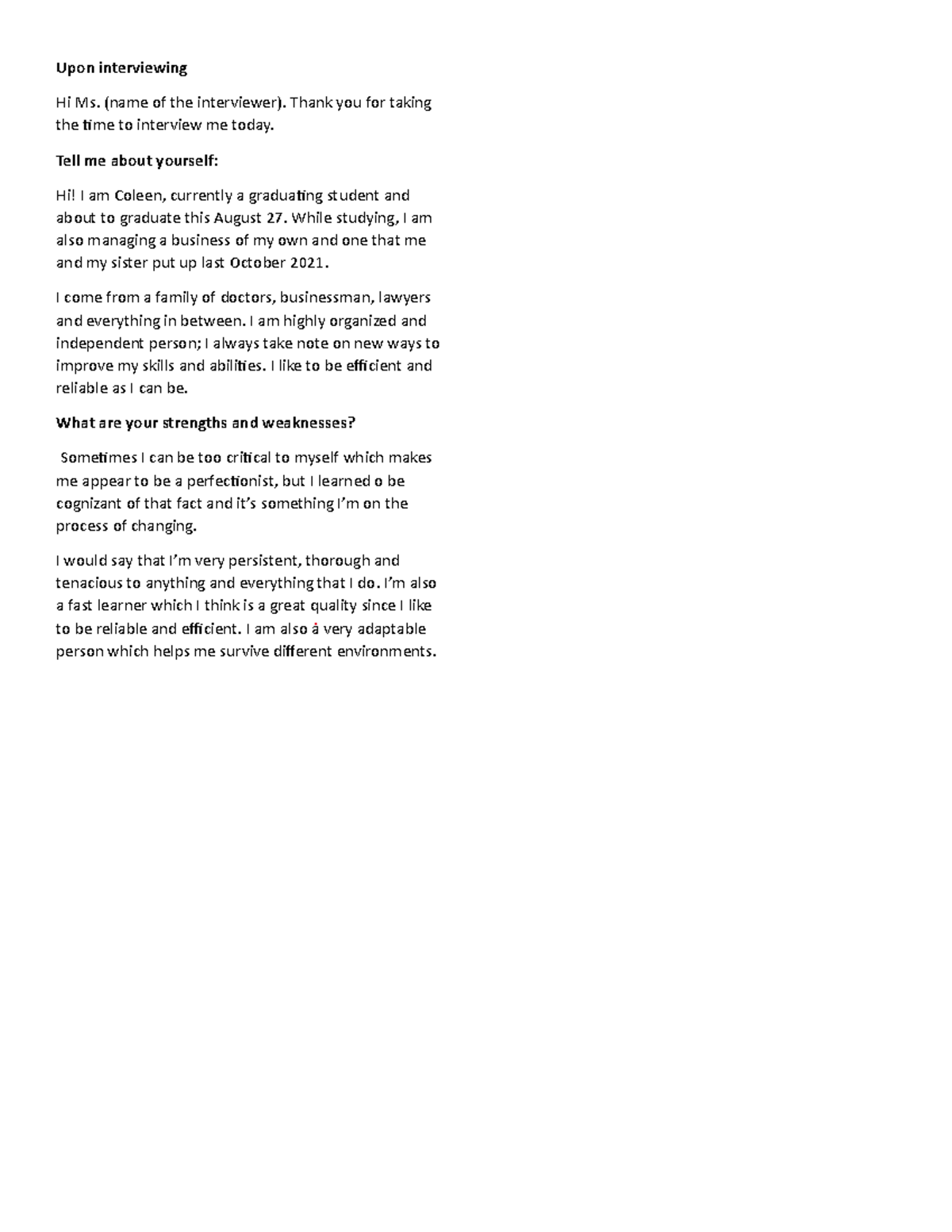**Screenshot of Interview Content on White Background with Black Text**

Upon Interviewing

Hi [Name of the Interviewer], thank you for taking the time to interview me today.

**Tell me about yourself**

Hi, I am Colleen. I am currently a graduating student and about to graduate this August 27th. While studying, I am also managing a business of my own, which my sister and I established in October 2021. I come from a family of doctors, businessmen, lawyers, and various other professionals. I am a highly organized and independent person. I am always seeking new ways to improve my skills and abilities. I strive to be as efficient and reliable as possible.

**What are your strengths and weaknesses?**

Sometimes, I can be overly critical. However, I would say that I am very persistent, thorough, and tenacious in everything that I do.